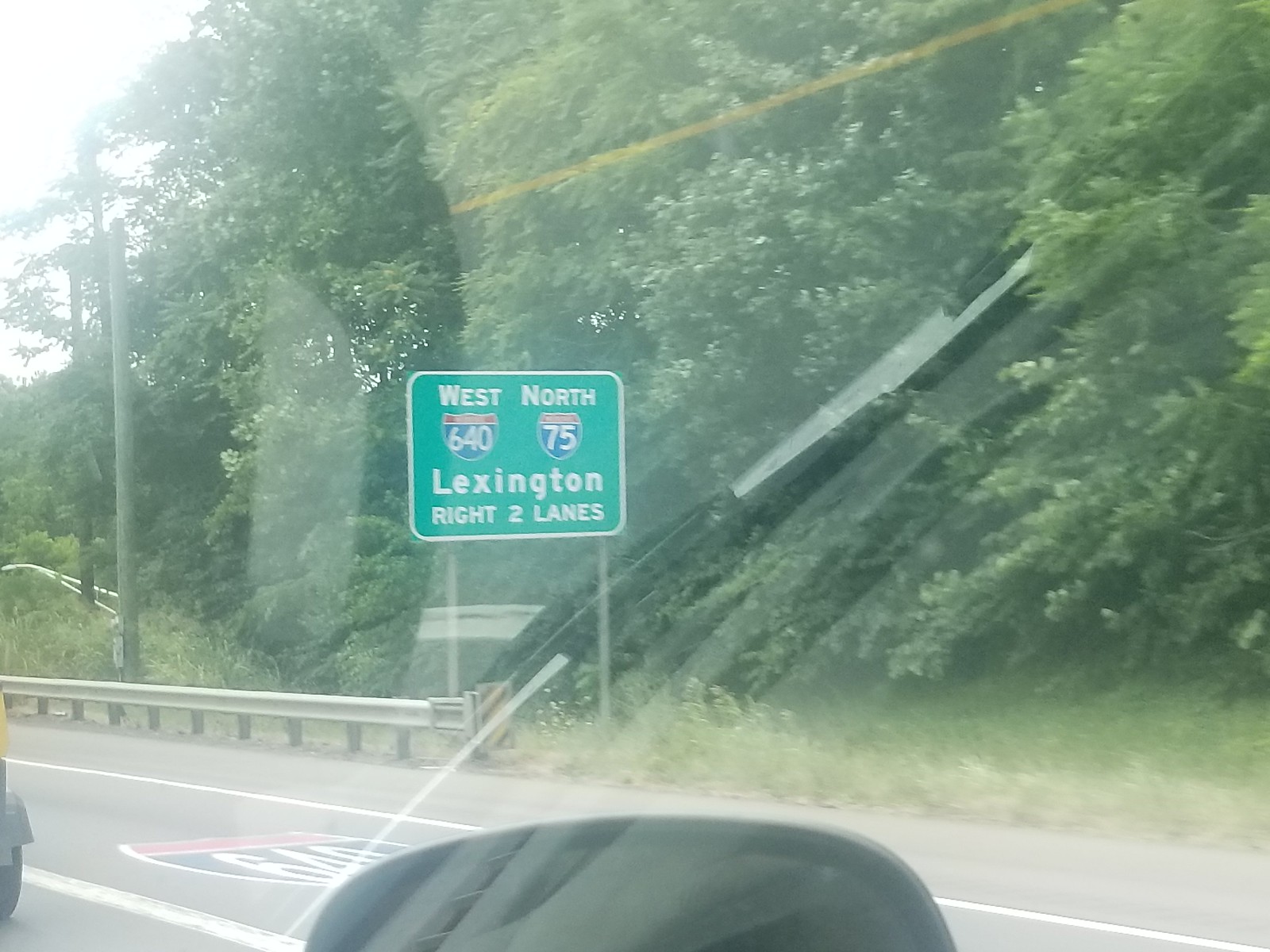This photograph captures a highway scene taken from the passenger side window of a moving vehicle. The image prominently features a road sign in the center, which indicates directions for West 640 and North 75, with a message in white font stating, "Lexington right two lanes." The highway guardrail extends from the left edge of the image to nearly the center, guiding the viewer's eye towards the sign. The background is dominated by a dense cluster of trees, partially shrouded by an overcast sky. The glare from the passenger side window is visible, adding a touch of realism to the scene. Additionally, the top portion of the passenger side mirror is seen at the bottom of the image, reinforcing the perspective that the photograph was taken from within a moving vehicle.